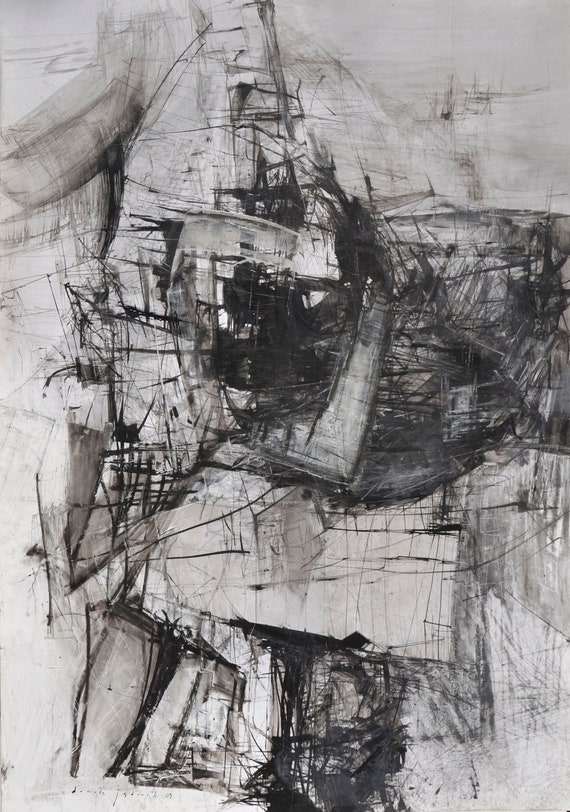This image depicts a black and white abstract artwork, characterized by a chaotic mix of colors and shapes that evoke a graffiti-inspired style. There are no discernible patterns or distinct imagery, just a dynamic blend of black lines and rectangular forms scattered across the surface. The background appears to be a white and grey, possibly resembling marble or polished granite, which contributes to the overall contrast and texture of the piece. The image showcases a variety of techniques, including streaking black lines, smeared grays, and shaded sections, some of which bear the marks of what might resemble smudging by fingers. The overall impression is one of disarray and intensity, with geometric shapes and scattered black blocks that occasionally suggest vague forms like a wrecked ship. Despite its chaotic appearance, the artwork’s lack of text and consistent shapes invites the viewer to interpret its meaning freely.